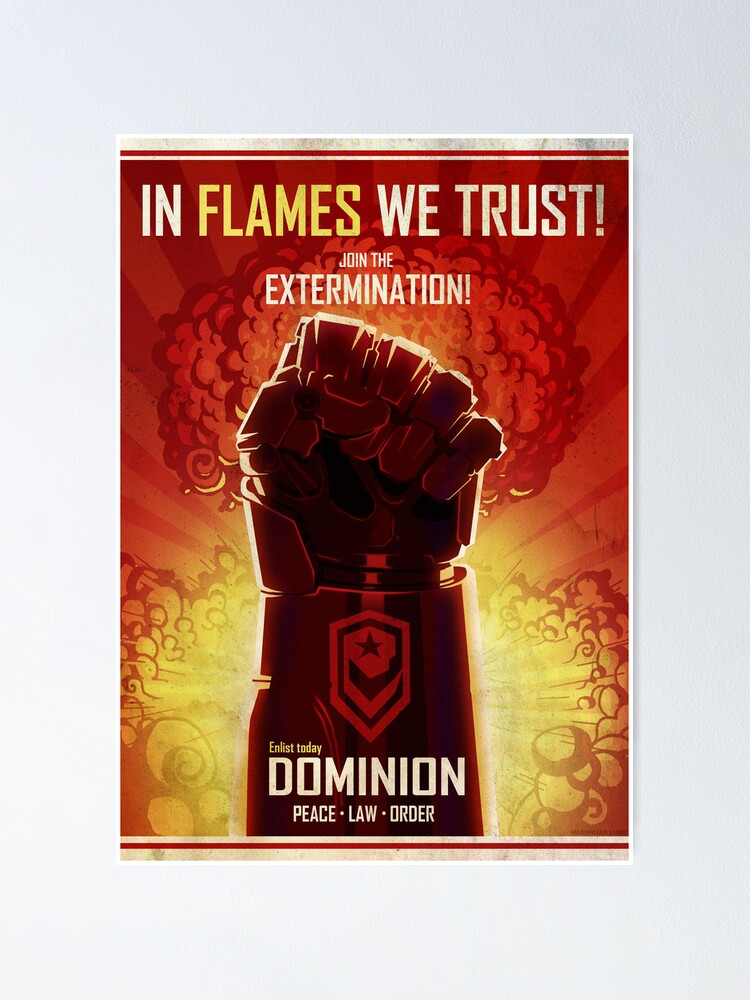The poster is a dramatic, propaganda-style advertisement for a video game, with a prominent theme of fiery destruction. The top half of the poster features a striking blend of red and yellow tones, depicting a massive explosion reminiscent of a nuclear mushroom cloud. At the top, bold white text reads "In Flames We Trust," with the word "flames" highlighted in yellow. Below this, smaller text states "Join the Extermination," with "Extermination" emphasized in larger font.

Central to the image is a large, dark, clenched fist extending upwards, resembling more of a robotic arm than human. The forearm bears a red shield-shaped emblem with a star at its center. Beneath the fist, the poster commands "Enlist Today" in dominant text, followed by the word "Dominion." Further below, in smaller text separated by dots, it promotes "Peace • Law • Order."

The overall design is aggressive and chaotic, with swirls of red and yellow flames enhancing the sense of urgency and conflict. A white border frames the entire image, adding to the polished look of a professional marketing poster.